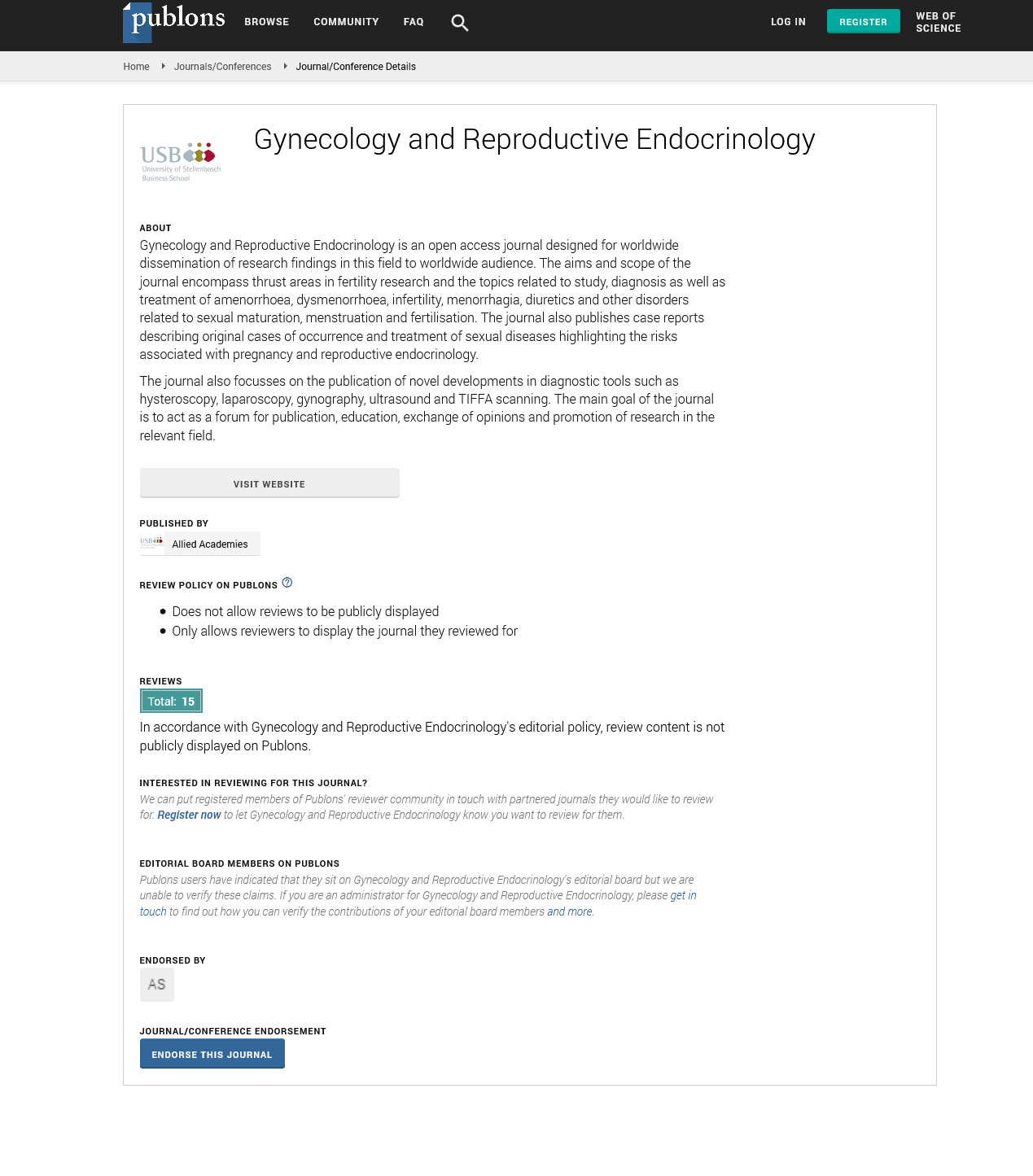The image depicts a webpage from the University of Stellum Broach Business School (USB), prominently showcasing an academic journal. At the top center, in the largest text on the page, the title "Gynecology and Reproductive Endocrinology" is displayed.

Below the title, a brief description explains that "Gynecology and Reproductive Endocrinology" is an open-access journal dedicated to the global dissemination of research findings within this medical field. The journal's aim and scope encompass vital areas in fertility research and address various topics related to the study, diagnosis, and treatment of conditions such as amenorrhea, dysmenorrhea, infertility, menorrhagia, diuretics, and other disorders linked to sexual maturation, menstruation, and fertilization.

Moreover, the journal includes case reports that describe original cases, occurrences, and treatments of sexual diseases, underscoring the risks associated with pregnancy and reproductive endocrinology.

At the bottom, there's a call-to-action button labeled "Visit Website," indicating that the journal is published by Allied Academies. 

Additionally, there's a note about the journal's review policy, emphasizing two key points:
1. Reviews are not allowed to be publicly displayed.
2. Reviews are only displayed for the journal they were specifically written for.